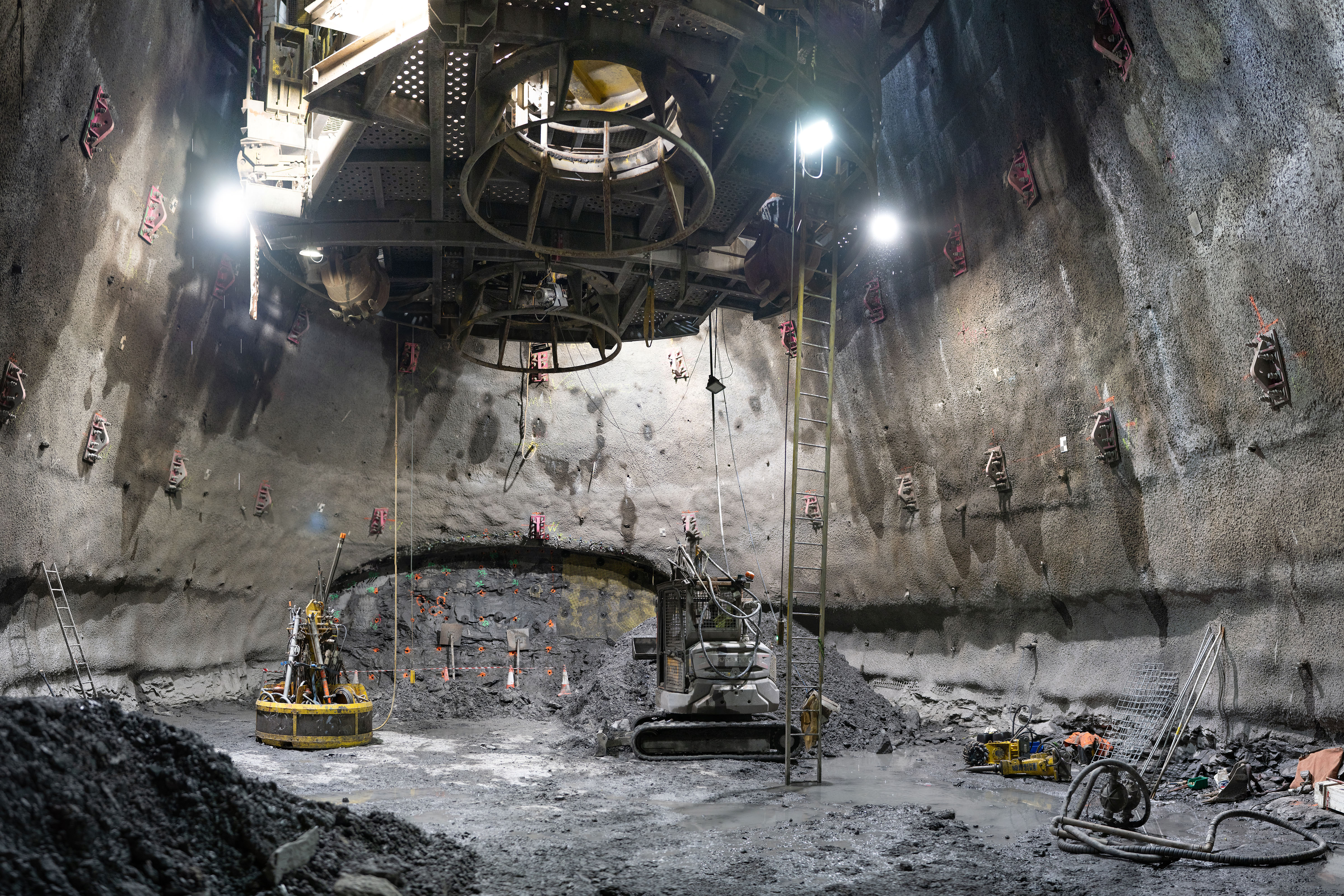The photograph captures the interior of a cavernous underground space, likely a mining operation, with walls carved out of stone in a sweeping, domed arch. The ground is littered with wet dirt, gravel, and multiple piles of excavated soft rock, especially prominent in the bottom left. Heavy excavation machinery is scattered throughout the scene, with particular focus on a large, gray and black vehicle with treads centrally positioned on the right. A yellow and gray excavation vehicle is also visible, along with various other pieces of equipment and rock piles. A tall ladder extends from the ground towards the upward-reaching domed ceiling, which features a circular shaft with a metal rimmed cage indicative of an elevator shaft. Multiple bright white lights illuminate the space from above. While the machinery appears actively engaged in the excavation process, no people are visible in this snapshot, adding to the impression of a large, industrious pit being methodically dug and shaped by the intricate assortment of machinery.